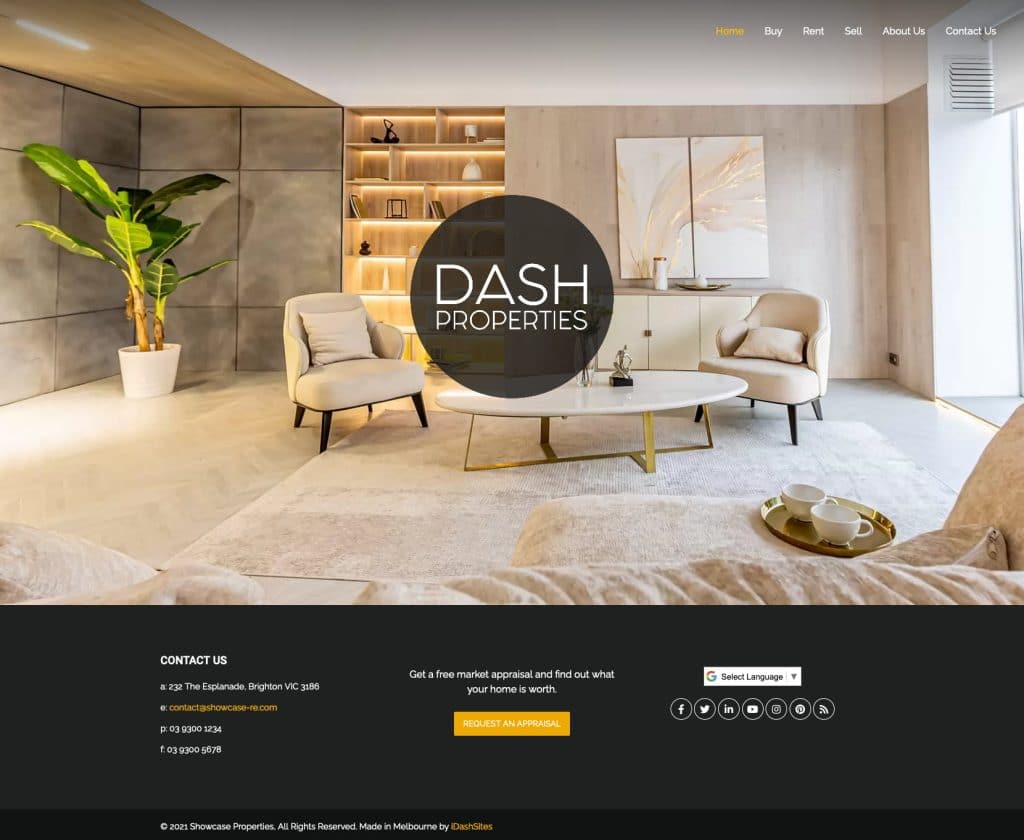**Caption:**
Screenshot of a Dash Properties webpage displaying a tastefully decorated living room. The room features a beige color scheme, a large plant on the left, and a big, sunlit window on the right. There are stylish pieces of art, decorative trays with vases, and matching chairs, suggesting a luxurious and well-designed space. The bottom third of the screenshot includes a black banner with contact information and a call-to-action button labeled "Request an Appraisal." Additionally, there are options for social media interaction, offering a comprehensive resource for prospective clients.